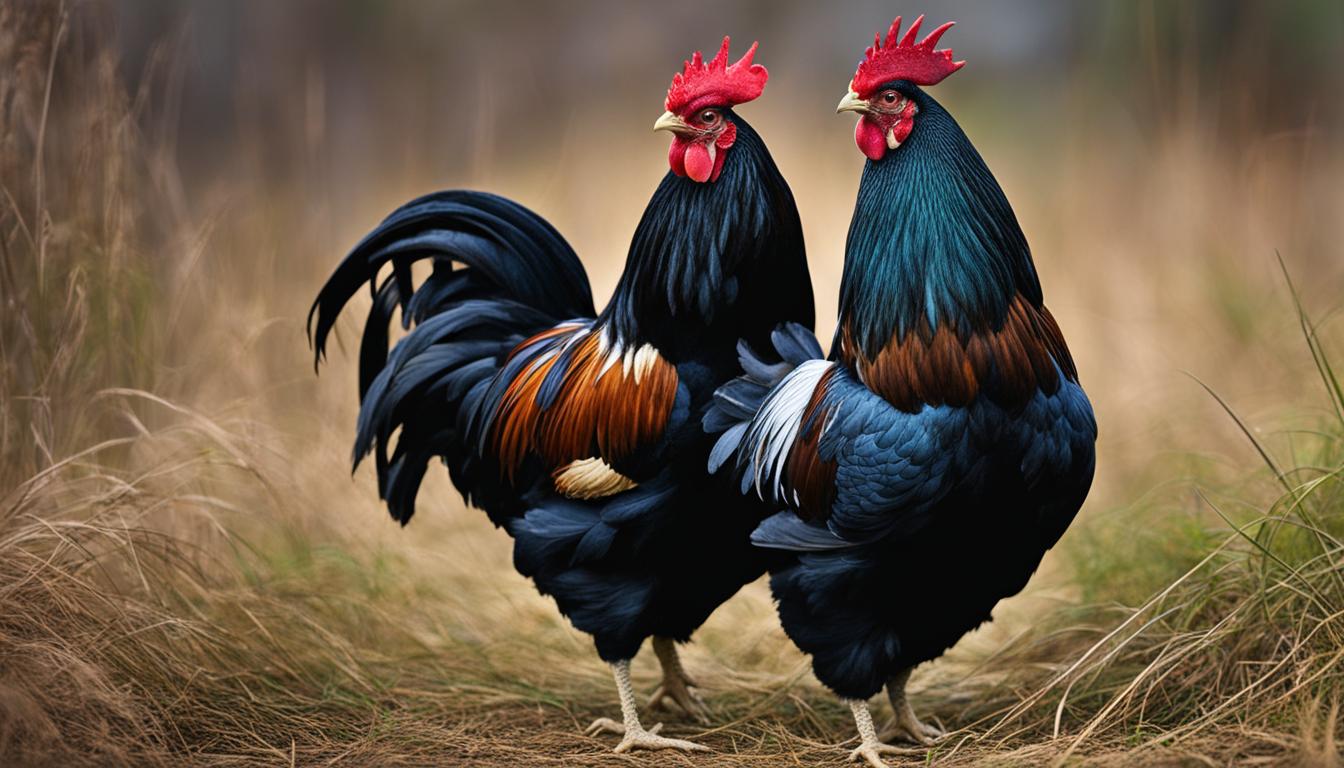This is a detailed painting of two striking roosters standing in a meadow primarily composed of grass and straw. Both roosters have a stunning turquoise or teal blue plumage with midnight blue accents. They are adorned with vibrant red combs on top of their heads and red wattles beneath their beaks, which are white. The roosters are both facing to the left, drawing attention to their contrasting feather patterns. The rooster on the right exhibits a patch of brown feathers where its neck meets its upper body, while the other displays a palette of brown, rust, and white feathers, with its tail feathers notably more erect. Their legs feature a light sand or cream-beige hue. The grassy foreground, rich in detail, is filled with predominantly brown, straw-like blades, while the background is intentionally blurred, emphasizing the birds as the focus of the artist’s work.